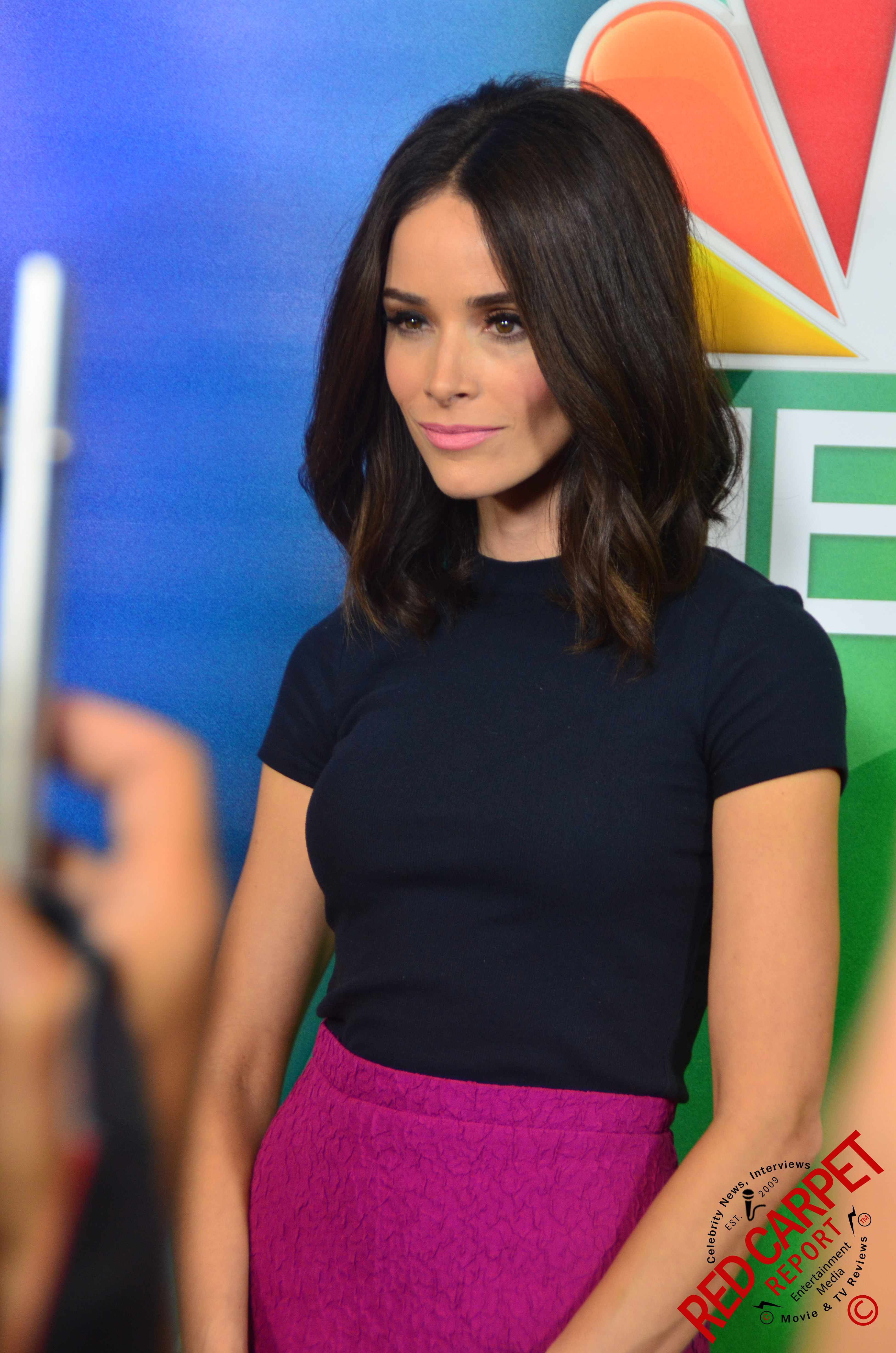The image portrays a young woman, likely a TV or movie star, standing from the waist up. She has straight, very dark brown or black hair that falls to her shoulders, complemented by dark eyelashes, dark eyes, and peaked lips. She is wearing a tailored black t-shirt with short sleeves and a pink or purple skirt. The background features a blue wall and the partial NBC logo with a peacock emblem, suggesting a connection to NBC News. In the lower right-hand corner, there is a watermark from "Red Carpet Report Entertainment Media," with text curving around it indicating "Celebrity News Interviews Established 2009 Entertainment Media Movie and TV Reviews." The woman is looking slightly to her left with a subtle smile. There is also a faint, blurry image of a photographer's hands holding a cell phone visible on the left side of the photograph.